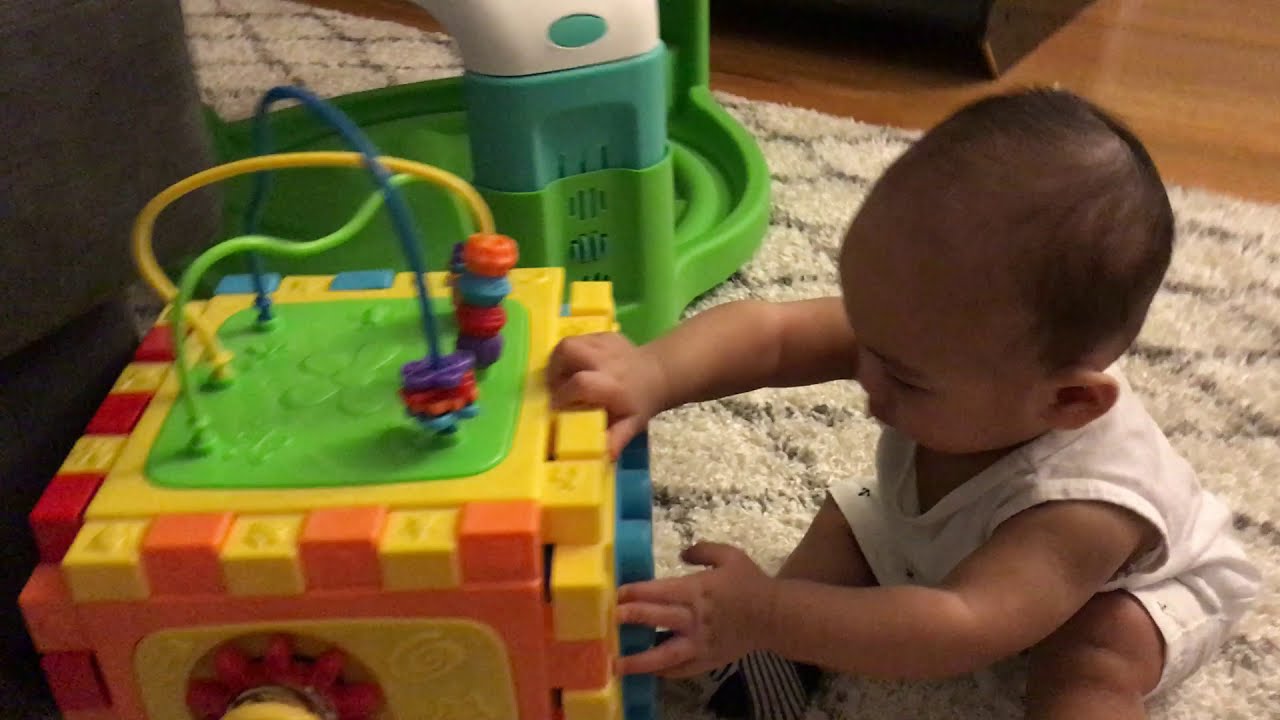In a warmly lit living room, a photograph captures an Asian toddler, around one year old, intently playing with an intricate toy. The child, with dark hair, is dressed in a sleeveless white onesie that reaches just above his knees. He is seated on a plush, gray rug adorned with diamond shapes, which stretches across a shiny hardwood floor. The colorful toy he is engrossed with consists of a yellow section that fits into an orange base, resembling a dovetail joint. Attached to the top of this toy are blue, green, and yellow cables with various weights, including shapes like flowers and circles, designed to slide along the rails. The toddler’s right hand firmly grasps the toy's top, while his left hand reaches out, fingers splayed, just touching the opposite side. His focused expression reveals his intrigue as he plays, surrounded by the cozy atmosphere of the living room. A mysterious green structure sits adjacent to the toy, contributing to the play environment, though its purpose remains unclear.